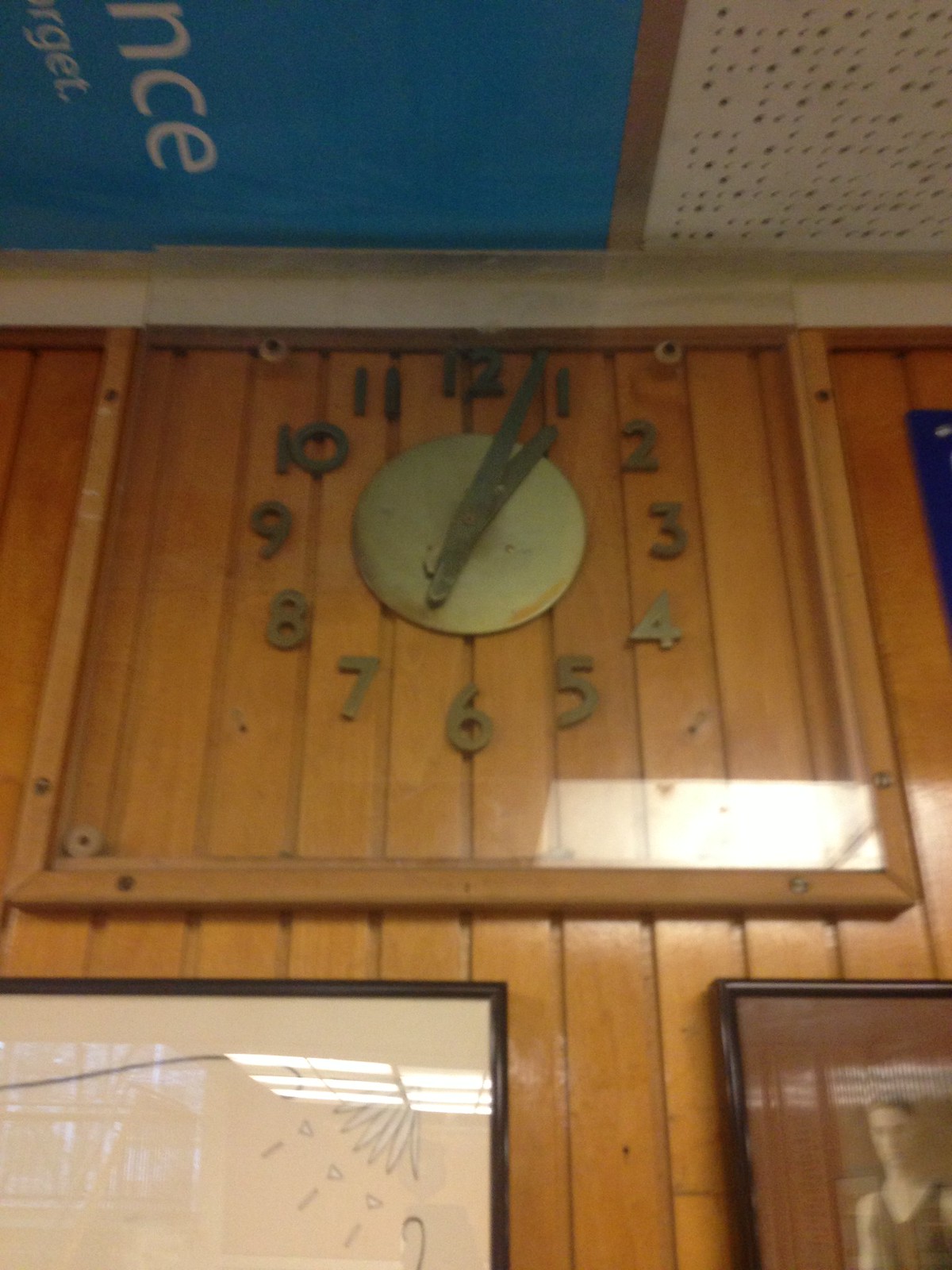The image captures a detailed close-up photograph of a clock mounted on a light brown wooden wall with vertical planks. The clock features a wooden frame and a piece of glass, giving the impression that it is almost floating within the glass. The hands of the clock are large and thin, and they rest on top of a circular piece of metal that is olive green, matching the color of the numbers, which are a darker shade of olive green. The numbers on the clock face range from 1 to 12, with some reflecting on the top part of the glass. The clock shows the time as approximately 1:03. 

Beneath the clock, two picture frames are hung on the wall. One of the frames contains a black-and-white photograph of a man wearing a sleeveless t-shirt set against a gray background. This frame has a black border and a brown mat. The second frame displays an abstract white image featuring etched patterns that resemble leaves with small triangles and rectangles, as well as a prominent blue line running through the design. The wooden wall also has white grouting visible between the planks, adding to the overall rustic aesthetic.